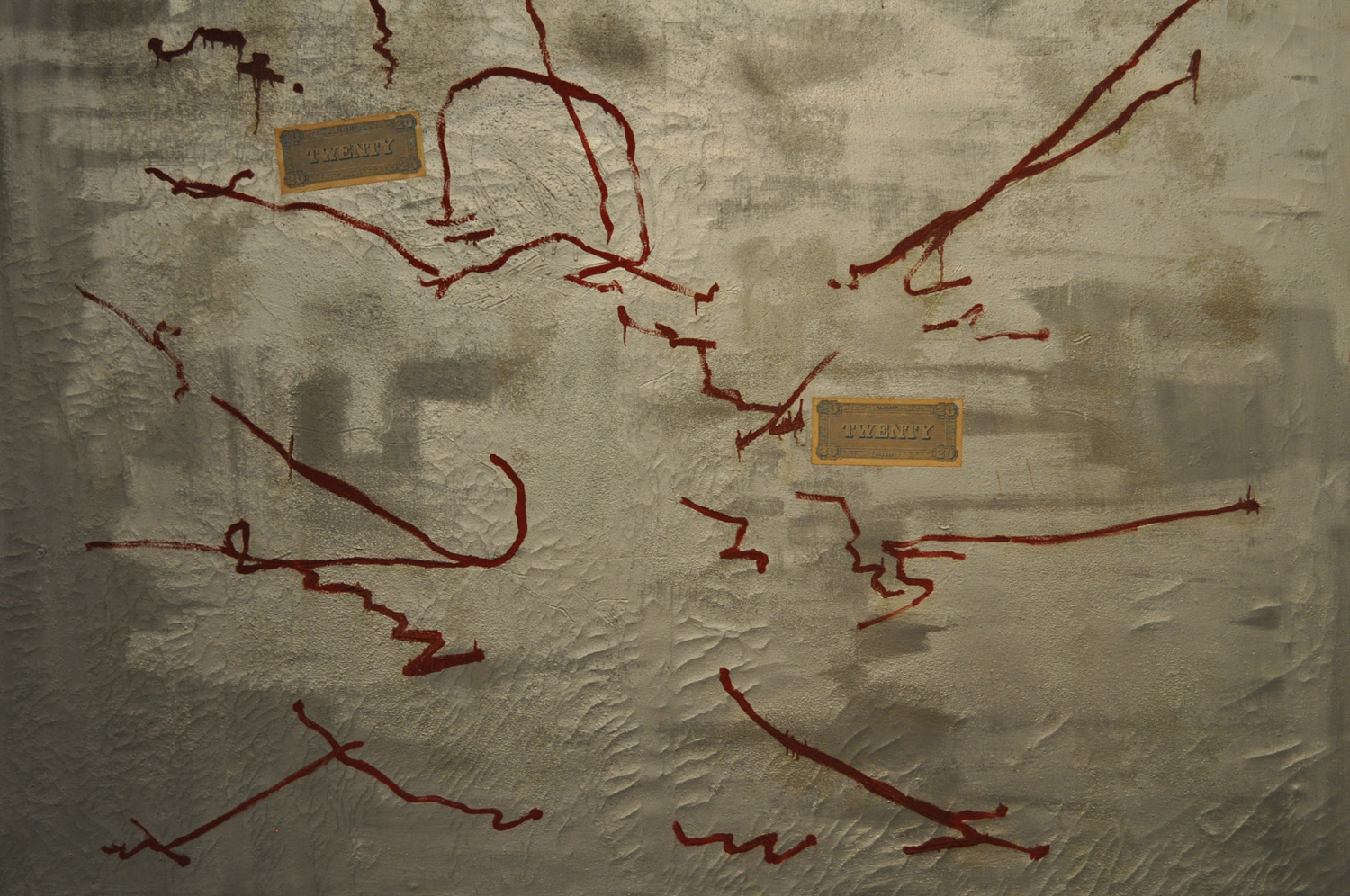The image showcases a photograph of a canvas artwork that occupies the entire frame. The canvas is predominantly beige, with gradients ranging from light to dark, especially on the outer left side. The surface of the canvas appears textured and wrinkled, with discernible cracks and shadowy areas, suggesting it might be either glued down or purposefully distressed. Erratic red lines, varying in thickness and shape, crisscross the canvas, created with a paintbrush or marker. Superimposed on this background are two fake orange-colored $20 bills, one taped in the top left corner and another slightly right of center. These bills feature the number 20 prominently in the center and smaller 20s encircled in each corner. Additionally, there seems to be some geometric or slightly transparent grayish areas adding to the visual complexity. The artistic elements combined create an abstract and somewhat chaotic composition.